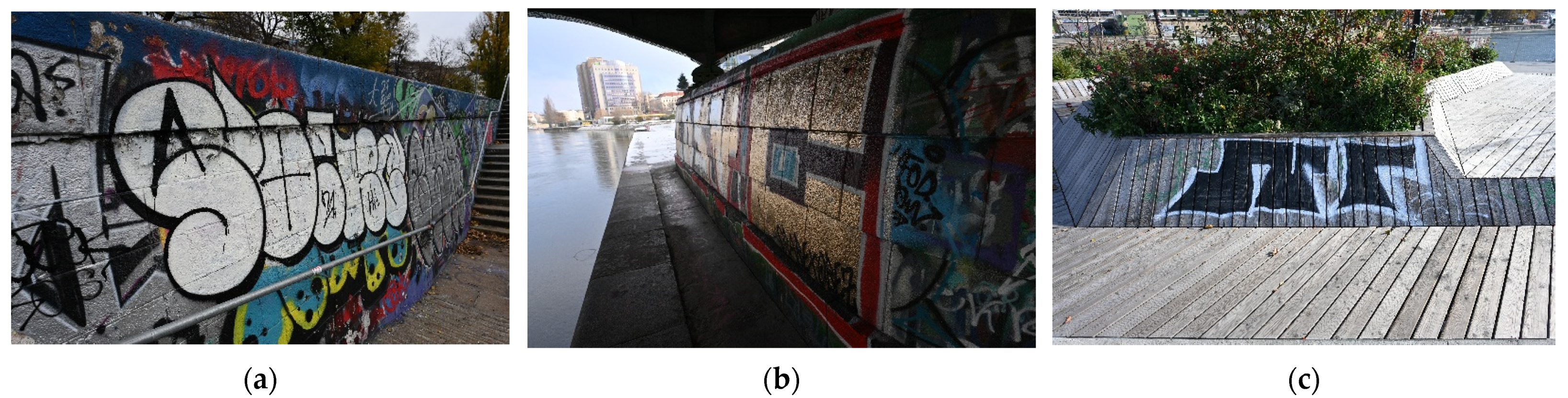The image showcases three distinct examples of graffiti labeled A, B, and C, all taken during the daytime. 

The first image, labeled A, features a wall adorned with predominantly white-lettered graffiti. The text starts with an 'S', followed by an 'O', 'I', and tapers off with ellipses before ending in a 'C'. The background is vibrant with hues of red, blue, yellow, cyan, and gray. There is also some gray text that's partially obscured. The scene includes a gray bar ascending a set of stairs on the left side.

The middle image, labeled B, depicts a dimly lit area under a bridge beside a riverway, with buildings visible in the background. The graffiti here is less discernible due to the lighting but includes a prominent gold letter 'C' with a black and red outline. There’s additional, harder-to-read graffiti surrounding it.

The third image, labeled C, captures graffiti on a wooden surface, featuring what appears to be three interconnected symbols: the first resembling an 'S', the second a variation of 'S', and the last resembling a '7'. The graffiti is rendered in bold black with a white stroke. This wooden structure seems to be part of a deck or stage with surrounding foliage, suggesting a possible pier or walkway setting.